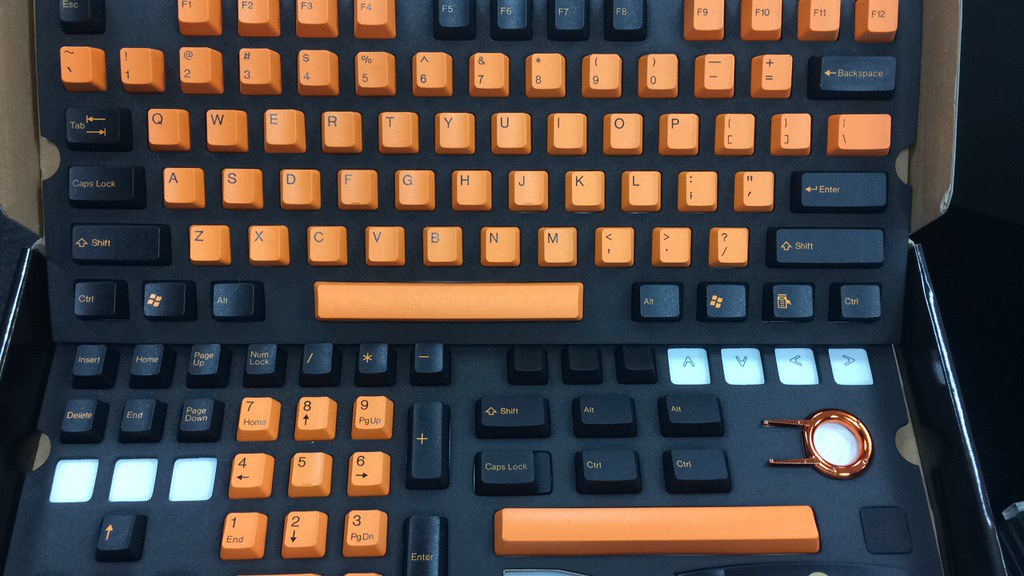This color photograph captures a unique, non-standard computer keyboard setup, broken into two separate units. Each keyboard has a black background with a combination of bright orange and black keys with orange lettering. The primary keyboard holds essential function keys such as Enter, Shift, Control, Backspace, and another spacebar, while the secondary keyboard features a numeric keypad along with additional keys like Shift, Alt, and Delete. To the bottom right, there's a golden keycap puller with a white center, beside what appears to be spare keys and three small white lights. The setup also includes a round symbol on the right side, covered in an orangey metallic cord extending to the left. The keyboards are placed on a slightly greyish background with hints of cardboard around the edges, suggesting they are inside a box or case. There are no other objects in the photo.